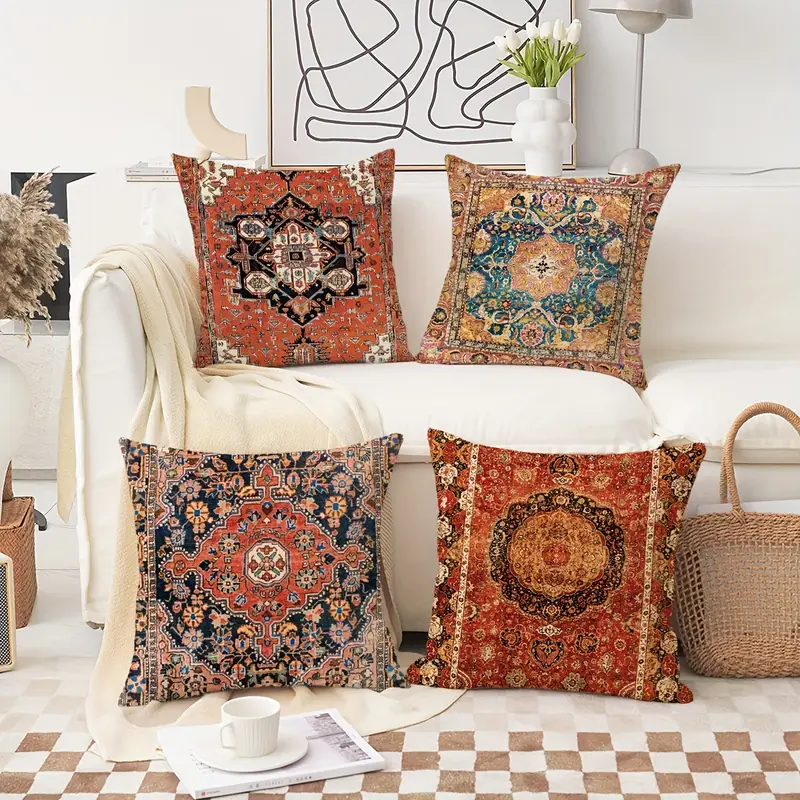This photo depicts a modern, minimally decorated living space centered around a beige fabric sofa adorned with a striking array of four Middle Eastern or Moroccan-style pillows. The pillows are intricately designed, showcasing rich, tapestry-like patterns in vibrant reds, oranges, golds, and bronzes. Two of these pillows rest on the couch while the other two are positioned against its base. The room features a checkered brown and white rug, reminiscent of a chessboard, upon which a book and a coffee cup with a saucer are carefully placed. Adding to the cozy ambiance, a yellow blanket drapes over the arm of the sofa and spills onto the floor near the pillows. A wicker basket and a checkered rug enhance the inviting aesthetic, and an abstract painting with black lines hangs on the wall above the sofa, completing the chic, modern look.